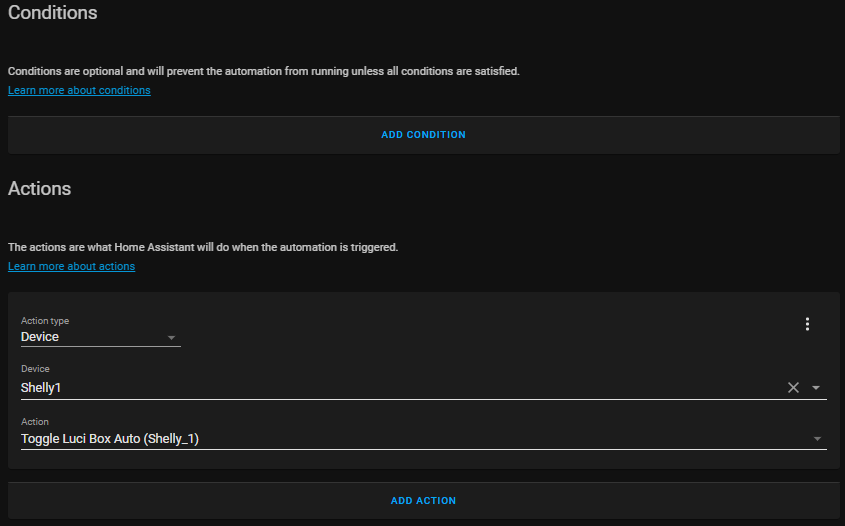In this image, we see a black screen with various sections and text inputs. Starting from the top left, the heading "Conditions" is prominently displayed. Directly below this heading, there is a small white sun icon.

Beneath the icon, in blue text, it says "Learn more about conditions," indicating a clickable link for additional information. Continuing downward, there is another blue link labeled "Add condition" positioned in the center of the screen.

Further down, the heading "Actions" appears, explaining that these actions will be executed by Home Assistant when the automation triggers. Following this section, there's another informational blue link saying "Learn more about Actions," which is also clickable.

Below this, the text "Action type" introduces a segment detailing the specifics of the actions. It lists "Device" as the action type, followed by the name "Shelly One." The action description reads, "Toggle Lucy Box (Shelly_one)," and there is a white horizontal line separating this segment from the ones above and below.

At the very bottom of the screen, in light blue text, there is an option to "Add action." The background of the image is predominantly black, with some dark gray elements at the bottom.

Overall, the image displays a structured and detailed interface for managing automation conditions and actions within a Home Assistant setup.